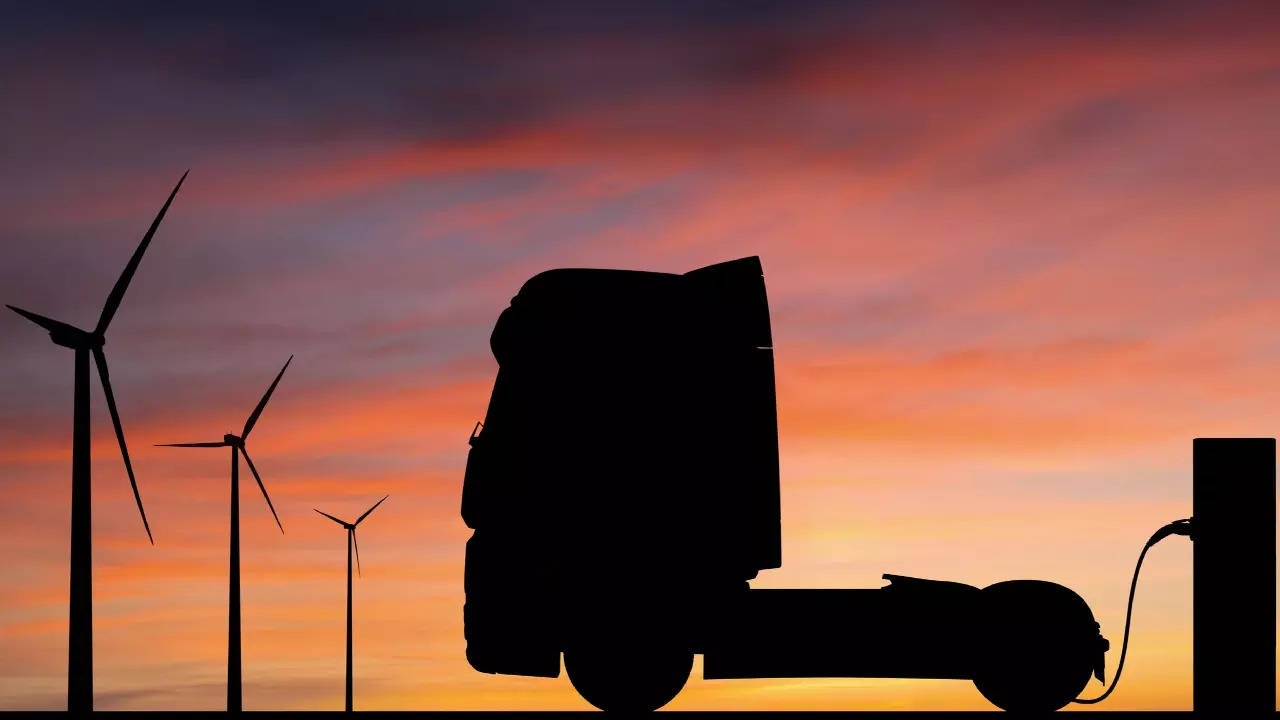The image features a digitally created scene of a vibrant two-tone sky with shades transitioning from peach and pink to a deep blue, particularly concentrated in the upper left corner. Below, the sky continues in these warm hues, interspersed with a touch of blue. Silhouetted against this colorful backdrop are three windmills on the left side of the image, aligned in a receding perspective from left to right, making them appear shorter as they move into the distance. Each windmill has three blades that are depicted in mid-rotation. In the center of the image, there's the dark silhouette of a semi-truck shown in a side view, oriented to the left. The truck is connected to a gas pump, which appears as a rectangular object on the right. The scene blends the movement of the windmill blades and the stillness of the truck, set against a visually striking, multicolored sky.